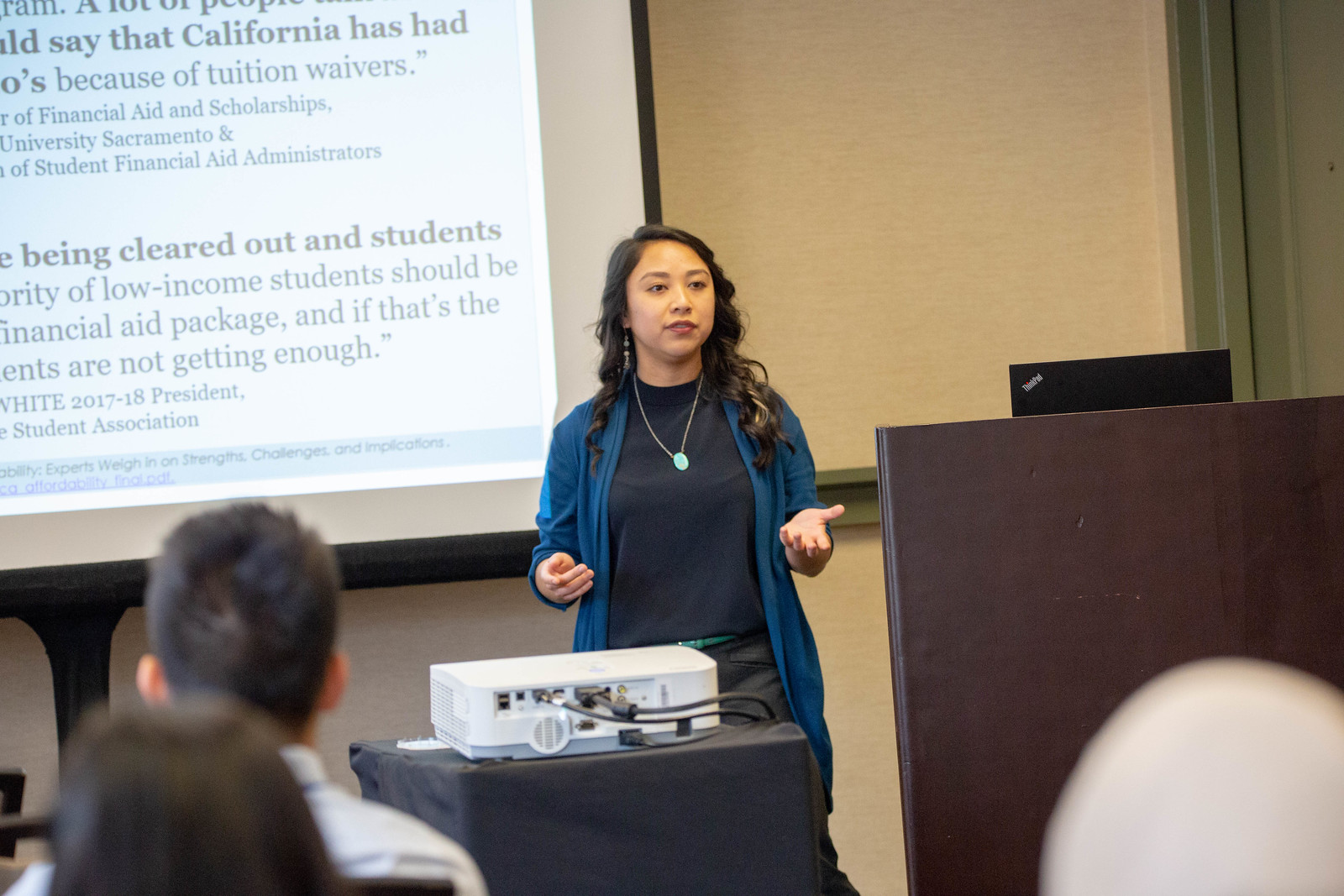The image depicts a horizontally aligned classroom setting with light brown walls and darker brown chair molding. A Filipino woman in her early 30s, with wavy, long brown hair, is giving an expressive presentation in front of an audience. She is dressed in a black shirt, a light blue or dark teal cardigan with a silver necklace that sports an oval-shaped pendant or greenish-colored gemstone. Her hands are raised as she speaks, and she stands near a brown podium to her right. 

To the left of the woman is a large projector screen displaying a partially visible PowerPoint slide. The text visible on the slide includes phrases such as "California has had," "tuition waivers," "financial aid and scholarships," "University of Sacramento," "student financial aid administrators," "being cleared out," and "students of low-income." However, most of the text is blurry or cut off. A white projector, placed on a small table with a black covering, projects the slide onto the screen. The audience includes an older gentleman with visible gray hair, seated in the front row, and a woman behind him with brown hair.